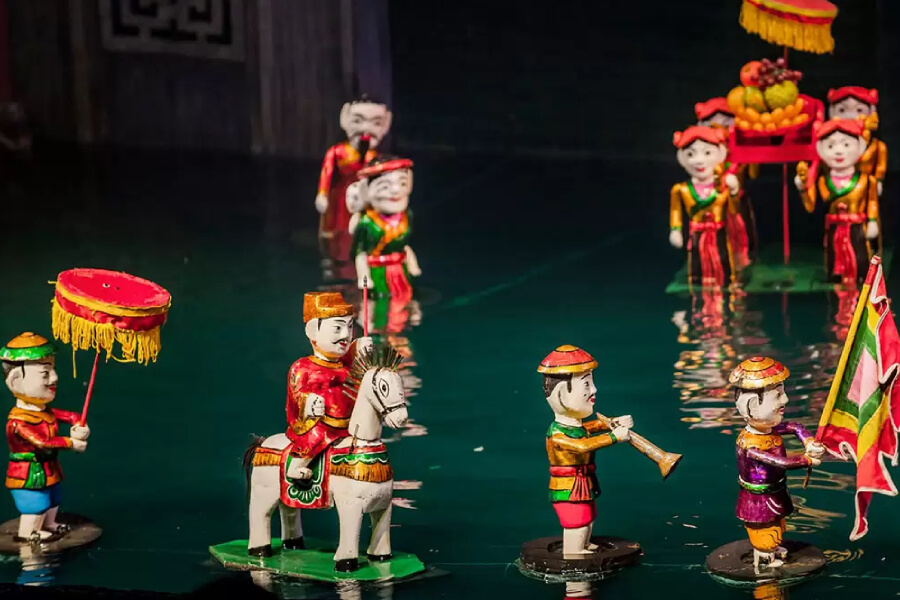This vibrant and detailed photo features a procession of hand-painted wooden Asian figurines set against a dark greenish-blue surface. At the forefront, a central figure is seated on a white horse, adorned in a red jacket and a flat-topped gold hat. To the left of this figure, another holds a red umbrella with yellow fringes, while further back, a group of women carries a cart topped with a bowl of fruit under an umbrella. Nearby, an older man in a red robe and a woman in a green and red robe add to the scene's rich tableau. The procession includes figures with sloping round hats; one blows a flared horn while another carries a flag with a red, yellow, and green motif. The image, characterized by its bright and vivid hues of red, gold, yellow, and purple, showcases a lively parade of intricately painted wooden toys, complete with musicians and spectators.